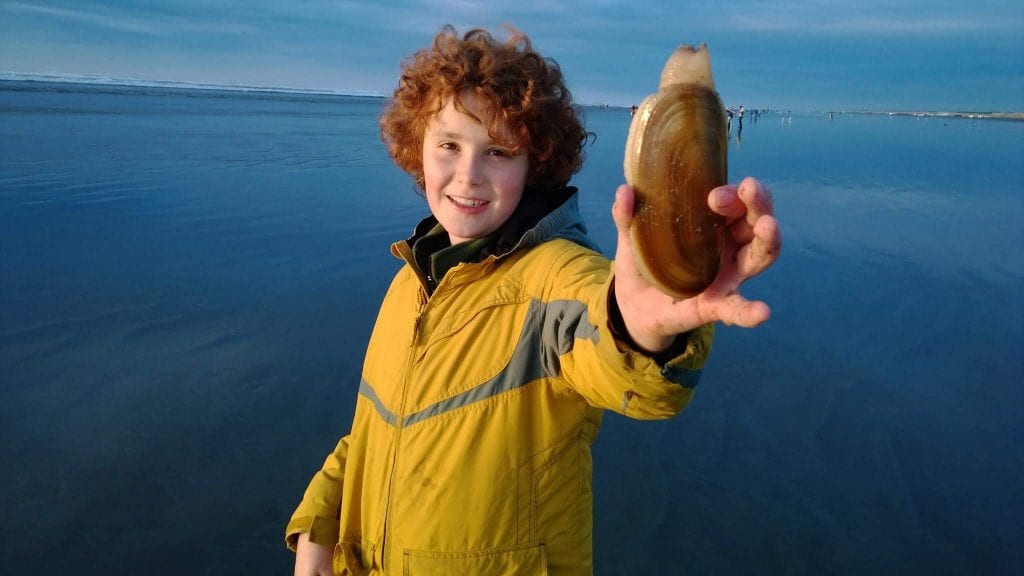A young boy with wild, curly red hair stands in the shallow, calm waters, smiling cheerfully at the camera. He is wearing a zipped-up yellow windbreaker jacket with a gray stripe across the chest, and a hood that is down. The boy holds a large geoduck clam in his left hand, displaying its shiny brown shell and whitish body. Behind him stretches a serene body of water merging with the horizon, where a blue sky with a few wispy, flat clouds meets the sea. There are also other people standing in the water in the background, suggesting the water is not deep. The scene is predominantly composed of various shades of blue, accentuating the tranquil seaside atmosphere.